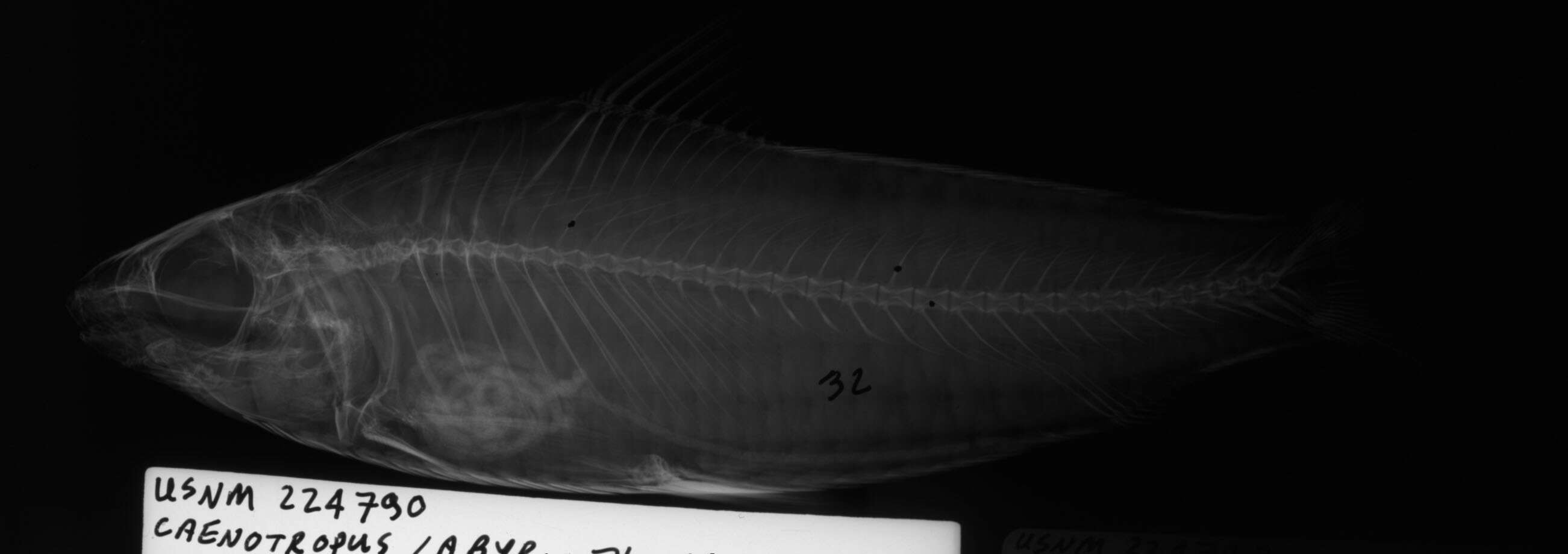The image displays an x-ray of a fish against a completely black background. The fish's head is positioned to the left, showing a distinct black section for its eye. The x-ray reveals the fish's skeleton, including its spine and the bones extending from it, in a lighter gray color. The outline of the fish's skin and some soft tissues, including faint details of its intestines and organs near the bottom of the body, are also visible. The darker regions of the fish's body, especially in the midsection and towards where the tail would be, contrast well against the dark gray of the fish itself. Although the tail area fades into black, most of the head and body are clearly seen. A small, black text "32" is visible in the middle of the fish. There is a white rectangular paper card with black handwritten text at the bottom of the image. The text includes "USNM 224790," "CAENOTROPUS," and partial text that seems to include "LARY," although the rest is cut off by the edge of the photograph. The overall image is in black and white.